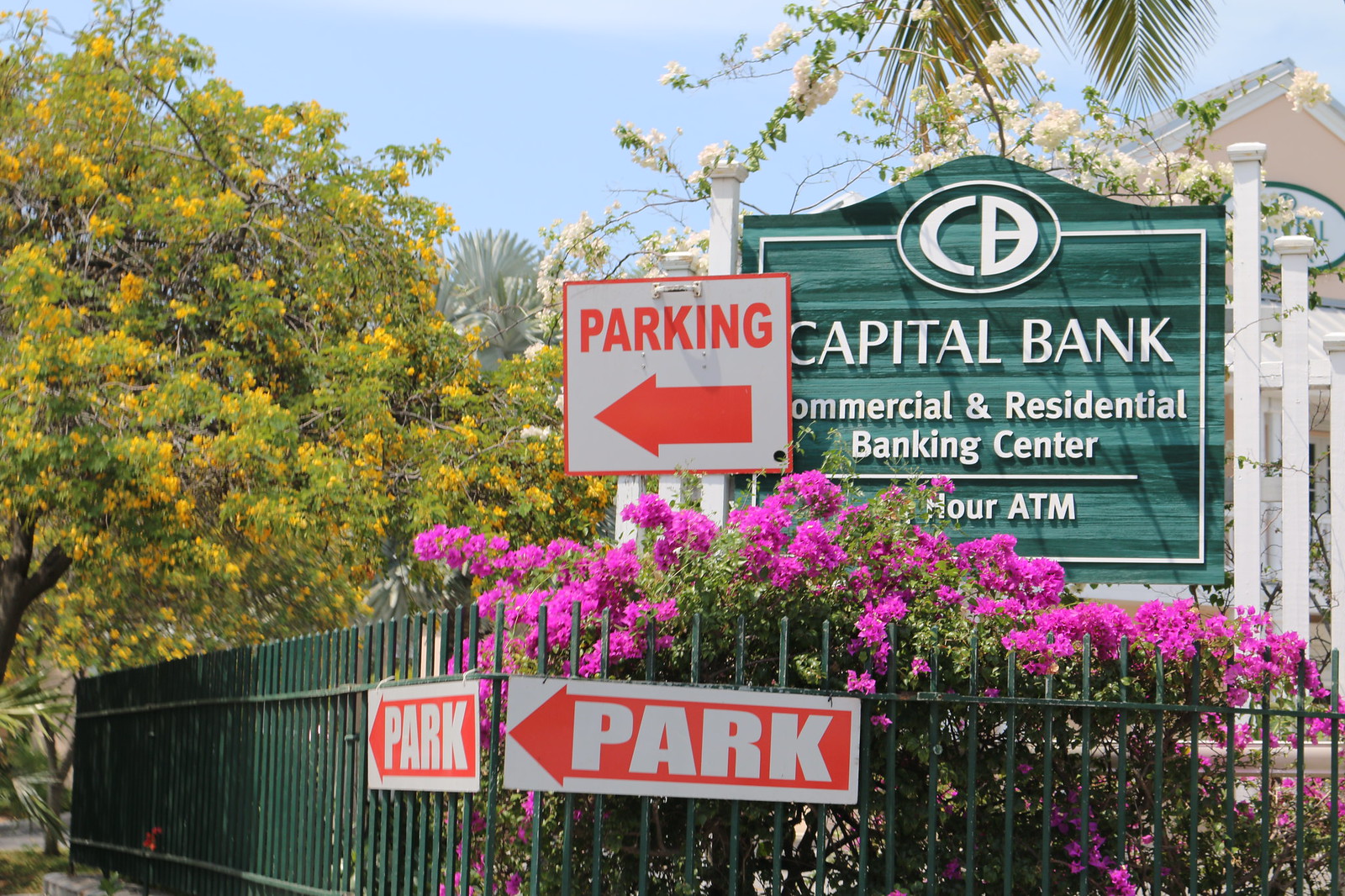This outdoor photograph showcases the Capital Bank location, which is prominently featured on a green sign with white text that reads "Capital Bank, Commercial and Residential Banking Center." The sign is mounted on a white post and sits behind a well-maintained green metal fence adorned with vibrant purple flowers. Above the Capital Bank sign, white flowers can be seen emerging, adding to the lush ambiance.

To the left of the main sign, there are multiple orange and white directional signs indicating "Parking" with arrows pointing left, suggesting the location of a parking area. The setting appears to be a well-maintained outdoor space, flourishing with blooming flowers and greenery, hinting at a spring or summer season.

In the background, the bank building itself stands with its yellow facade and white roof, surrounded by an array of trees, including palm trees positioned towards the back. The entire area exudes a neat and well-cared-for atmosphere, enhancing the welcoming appearance of the Capital Bank facility.